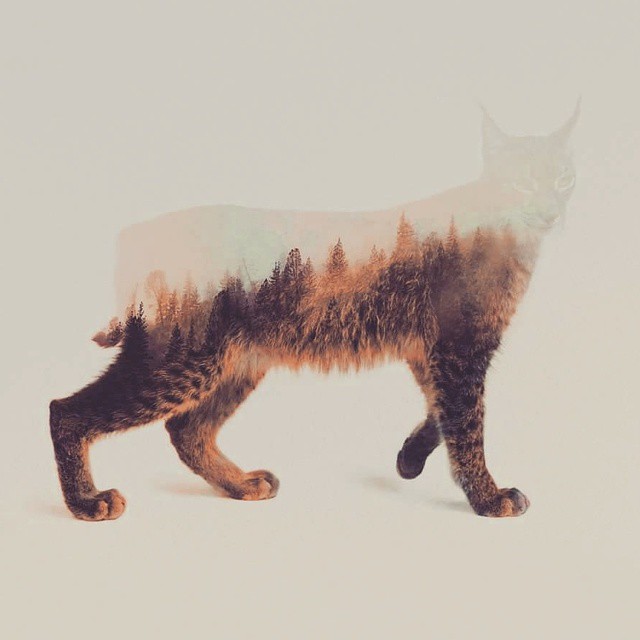The image depicts a striking artistic rendition of a lynx cat, blending realism and abstract elements. The background of the piece is a neutral tan or beige, providing a subtle contrast to the focus of the image. The cat, standing on all four legs, displays fur in shades of brown, black, reddish, and white. Its pointed ears and keen eyes are finely detailed, while the head and upper body gradually fade into ghostly silhouettes. This ethereal blending gives the impression that the top portion of the cat morphs into a forest of trees, creating a seamless transition between the animal’s fur and the arboreal forms. The paws and legs are distinctly visible, with the front left paw slightly raised off the ground. The tail’s tip can be subtly traced amidst the fading colors. The artwork masterfully integrates the physical and natural worlds, making the cat appear as though it is simultaneously a part of the forest it inhabits.